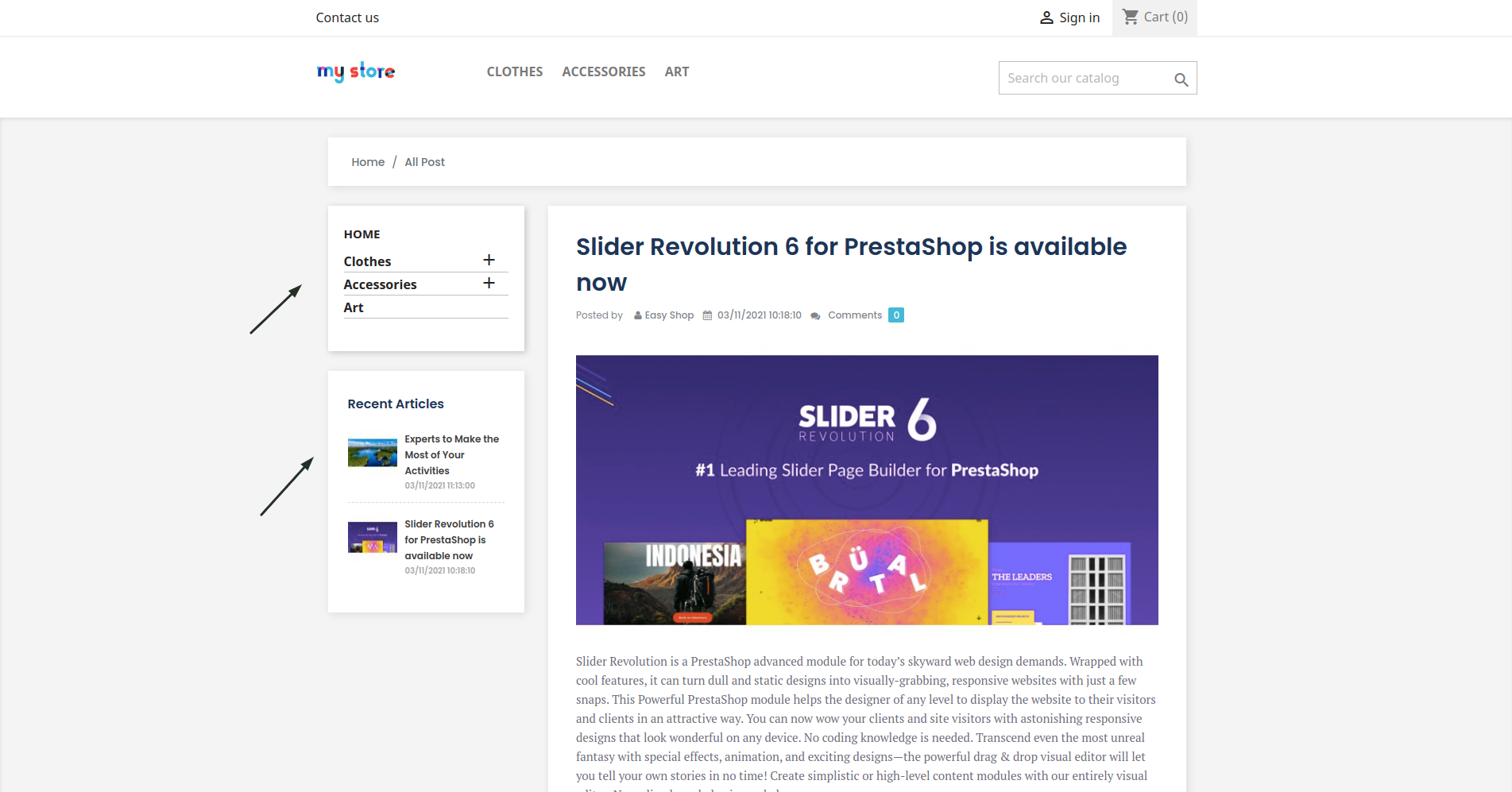The image showcases a webpage from a blog dated 2021. The page has a landscape orientation, appearing wider than it is tall. This particular webpage, viewed on a computer, belongs to a site named "My Store."

In the upper left corner, there's a "Contact Us" link, while the upper right corner features links for "Sign In" and a shopping cart icon. The "My Store" logo, characterized by a patchwork of colors, suggests a vibrant brand identity.

The navigation bar contains menu options for "Clothes," "Accessories," and "Art," alongside a search bar reader labeled "Search Our Catalog." Beneath this, a wide rectangular section displays the breadcrumb "Home / All posts," indicating the user's navigation path.

On the left side of the page, there are two prominent boxes, each marked with a black arrow pointing up from the left. The first box lists categories: "Home," "Clothes," "Accessories," and "Art." The second box highlights recent articles, linking to posts titled "Experts to Make the Most of Your Activities" and "Slider Revolution for PrestaShop is Available Now."

The larger main content area on the right showcases the selected post, "Slider Revolution 6 for PrestaShop is Available Now," published by Easy Shop on March 11, 2021 (noted as 03/11/2021), three years prior to the current date. The article heading is displayed on a large purple rectangle, emphasizing "Slider 6 Revolution: Number One Leading Slider Page Builder for PrestaShop." Three images are positioned beneath the heading, followed by a paragraph of text.

Overall, the website appears to sell various products, including clothing, accessories, and art, while also featuring informative blog posts.